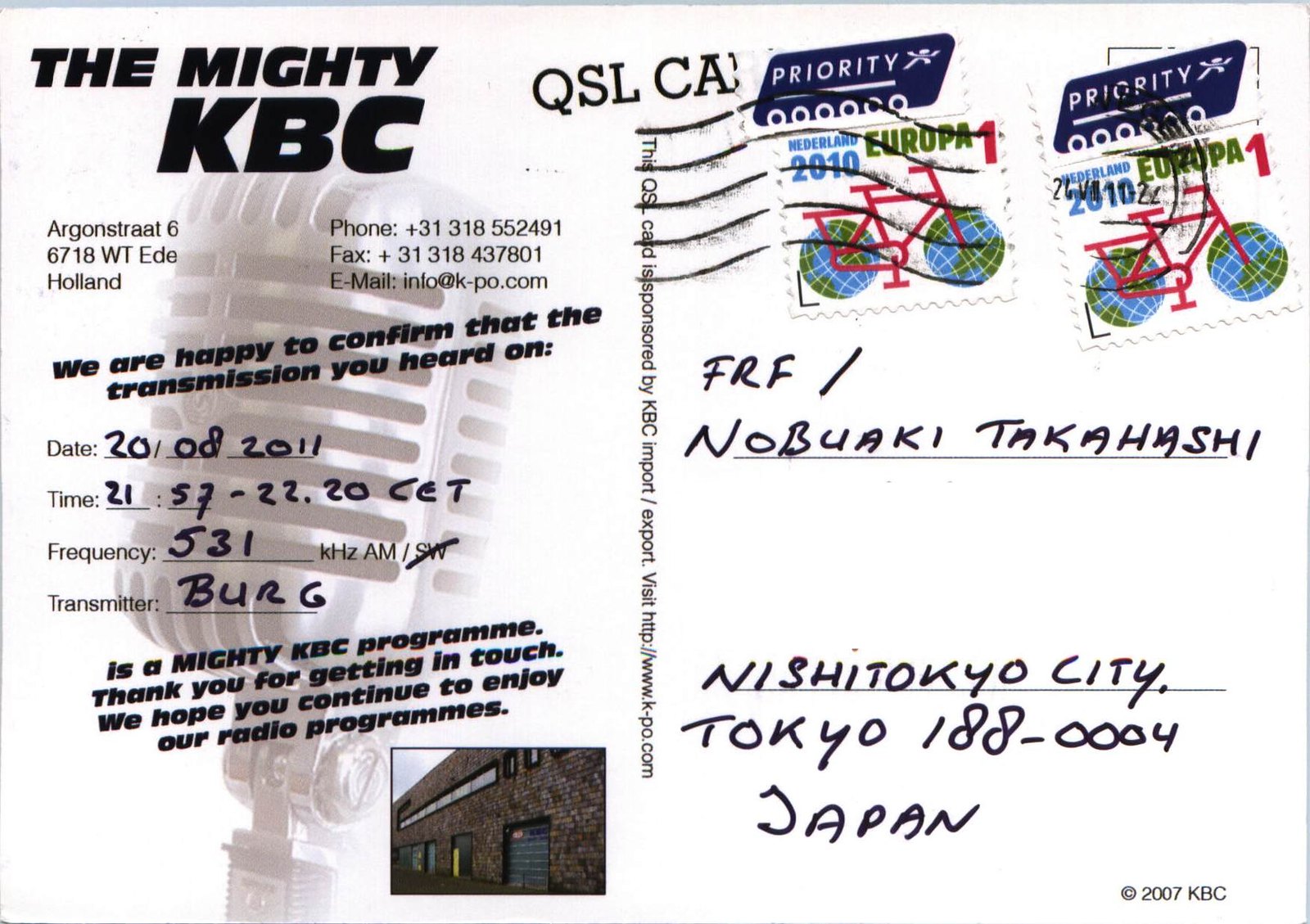The image depicts the back of a reception confirmation postcard divided into two sections. On the left side, there is a heading that says "The Mighty KBC" followed by their address: Argenstrat 66718 WTEDE, Holland, with contact details including phone number 31318552491, fax number 3138437801, and email info@k-po.com. A message underneath reads: "We are happy to confirm that the transmission you heard on date 20.08.2011, time 21:57 to 22.20 CET, frequency 531 kHz AM, transmitter Berg, is a Mighty KBC program. Thank you for getting in touch, we hope you continue to enjoy our radio programs."

The right side features the recipient's information including the name "FRF/Nobuke Takahashi," and the address: Nishikayo City, Tokyo, 188-0004, Japan. There are also stamps that are postmarked, indicating its mailing journey.